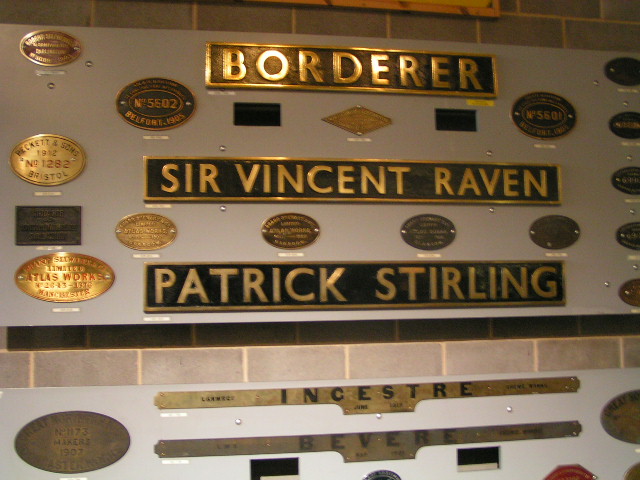This image depicts a series of gold-plated plaques with black backgrounds, mounted on a tiled wall. At the top, a large rectangular plaque features the word "BORDERER" in block capital gold letters. Below this, there is another rectangular plaque with the name "Sir Vincent Raven" also in gold letters on a black background. Underneath this, there are four smaller plaques, followed by another large rectangular plaque with the name "Patrick Sterling" flanked by smaller, belt buckle-sized plaques on either side. Surrounding these plaques are various emblems, mostly oval and rectangular in shape, all adorned in gold and black. Additionally, another white-bordered section below features plaques with the words "Ancestry" and "Bevere" in gold lettering. The image showcases a rich display of meticulously arranged, gold-plated plaques and emblems against a structured tiled wall background.